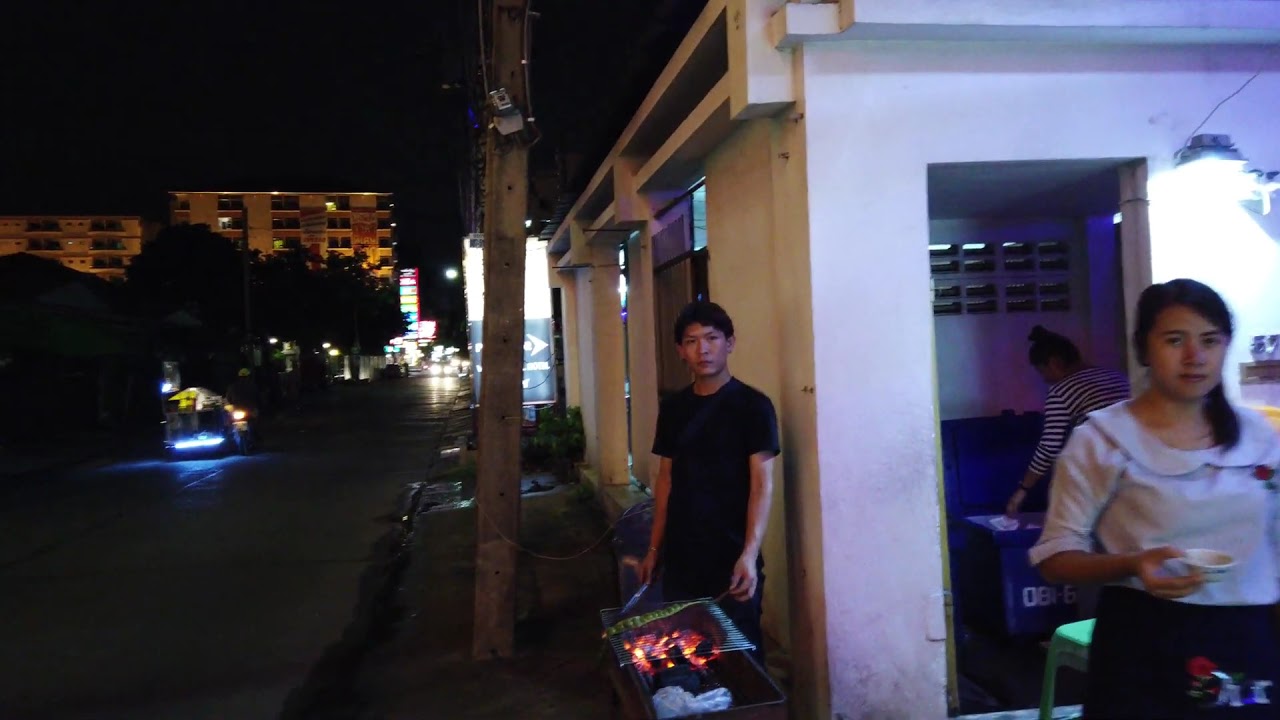The nighttime photograph captures a busy roadside restaurant scene in a city. In the lower right corner, a woman with black hair, tied up, wearing a white blouse with a red rose and a black skirt, stands holding a cup, possibly indicating she is a waitress preparing to place it on a table. Slightly behind her, inside the white cement building with bright white lights, is another woman with black hair and a black and white striped shirt, standing in a small area that appears to store linen. Centrally positioned, a young man with short black hair, dressed in a black t-shirt and black pants, is grilling fish and other items on an older-style metal grill set up outside the restaurant. He looks directly at the camera. The restaurant stretches down the major street visible on the center-left of the image, where a bus with headlights on is approaching the camera. The background features an apartment building lit up in brown, with rows of trees in front, and other city lights and vehicles fading into the distance.